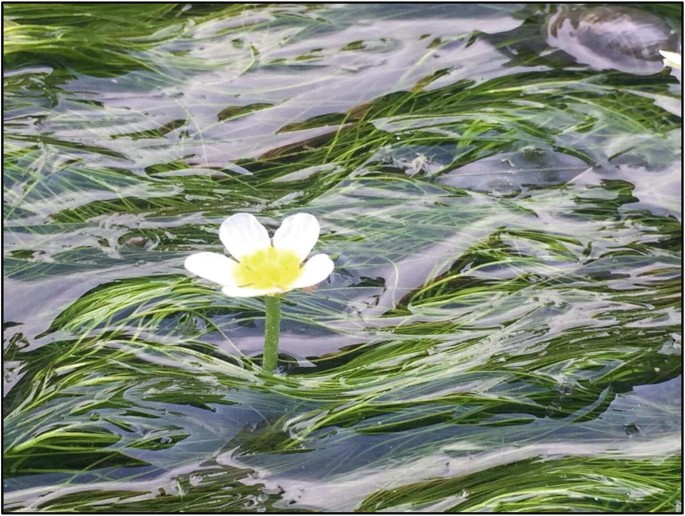This horizontally oriented image, which appears to be a realistic photograph, captures an outdoor scene during the daytime, suggested by the good lighting and natural outdoor elements. The picture is taken from about 10 feet above the surface of rippling water, angled slightly downward to showcase its detailed composition. The water is a deep blue mixed with white reflections of sunlight, and it has gentle waves moving over a bed of green seagrass. The seagrass, looking clean and untangled like long strands of fine green hair, ranges from one to three feet in length. Amidst this vibrant aquatic setting, a single, prominent flower rises out of the water, positioned towards the middle to left side of the frame. This flower features a green stem supporting five white petals that surround a bright yellow center. The flower stands out distinctly against the dynamic backdrop of shimmering water and swaying grass. The edges of the image are black, adding contrast to the vivid scene. While it might be a natural photograph, there's a possibility it has been digitally edited, although it convincingly portrays a natural aquatic environment.